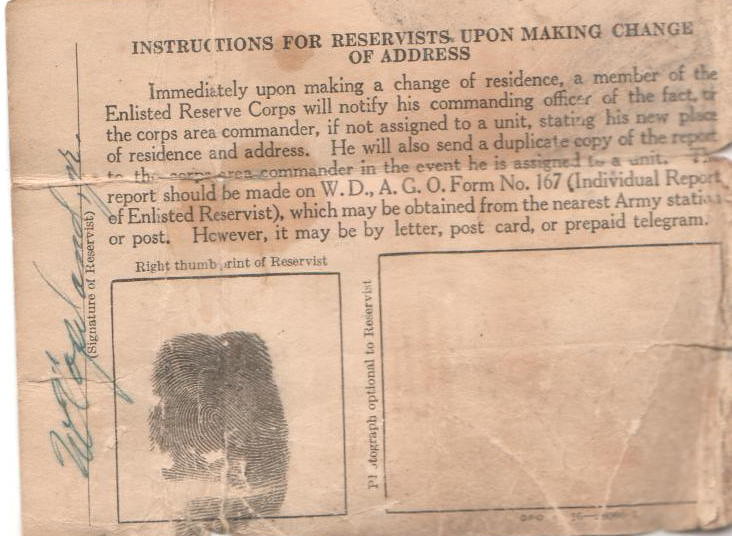The image features an old, aged legal document that resembles a newspaper clipping but is, in fact, a form titled "Instructions for Reservists Upon Making Change of Address." The document is specific to members of the enlisted reserve corps and contains detailed directives for notifying their commanding officer upon changing residence. The instructions specify that notification can be made via WDAGO form number 167, a letter, postcard, or prepaid telegram. The form includes a paragraph of text at the top, providing these instructions. 

On the lower part of the form, there are two marked sections. The left section contains a right thumbprint, while the right section, vertically aligned with the thumbprint, has a space for a signature written in blue ink. Additionally, beneath the paragraph, there are lines indicating spaces for the reservist’s signature and thumbprint, and a note that a photograph is optional. The document is monochromatic with shades of black, white, gray, and blue.